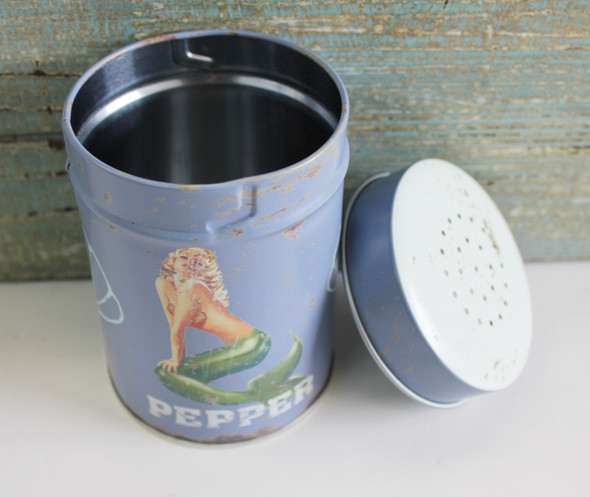The image depicts a vintage-style tin container used for pepper, characterized by its weathered appearance and distressed marks. The tin, which is approximately three to four inches tall, has a worn, white-blue or light blue exterior that might appear light purple or steel gray to some. A prominently featured, seductively posed mermaid with long blonde hair, green fins, and a potentially topless appearance (possibly wearing a seashell bra), adorns the side of the container. Her hands rest on her knees, and she leans slightly to the left while facing forward. Below the mermaid, the word "PEPPER" is printed in bold, white capital letters. The lid of the container, which has holes for dispensing pepper, is unscrewed and leaning against the right side of the tin. This entire scene is set against a background of weathered, teal-colored wooden walls with a peeling paint effect, and the container rests on a white surface.